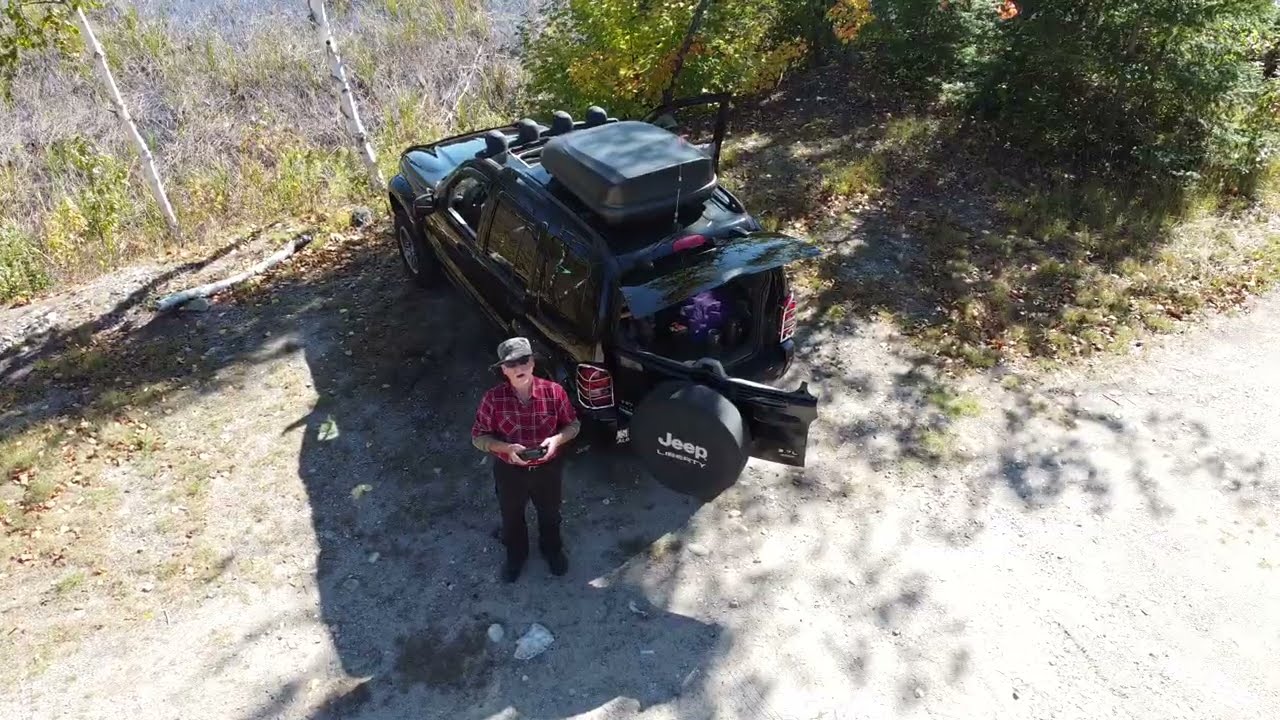The image captures an outdoor scene of an older man in his 60s, standing in a rural mountain range area during the daytime. The man is looking up, possibly at a drone, holding a black controller in both hands. He is dressed in a red plaid button-down short-sleeve shirt, black pants, black shoes or boots, sunglasses, and a green baseball cap. He stands on dirt and gravel, next to his parked black Jeep Liberty, which has a traveling gear rack on top. The Jeep is positioned with its back end towards the observer, and its rear door, bearing the Jeep logo and spare tire, is open. The setting features a mix of trees with green and yellow leaves, some bare trees, and various grasses and weeds, indicating a hillside or campground area with a slope. Sunlight casts shadows on the ground, enhancing the rugged and serene landscape.